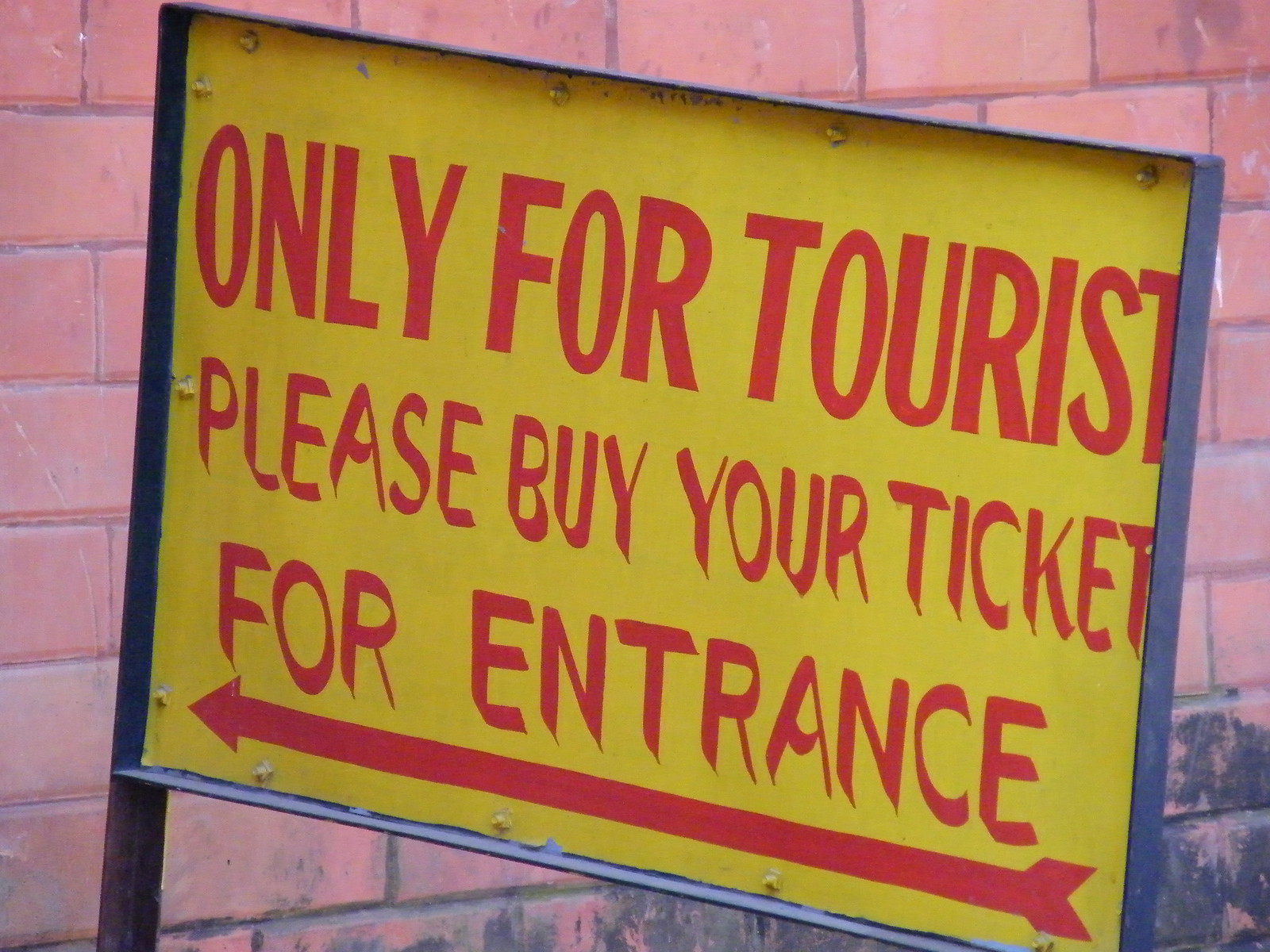The image depicts a large yellow rectangular sign, framed in black metal with rivets along the edges, bolted to black poles on each end. The sign stands outside the entrance of a building, angled slightly from the perspective of the photo. The background features a lightish-red brick wall with darker, maroon-colored grout, and noticeable black stains splashed towards the bottom right corner. The sign's text, which is in large, all-capital red letters, reads: "ONLY FOR TOURISTS," "PLEASE BUY YOUR TICKET," and "FOR ENTRANCE," with a long red arrow pointing to the left. The lettering appears hand-painted and is in two different fonts.